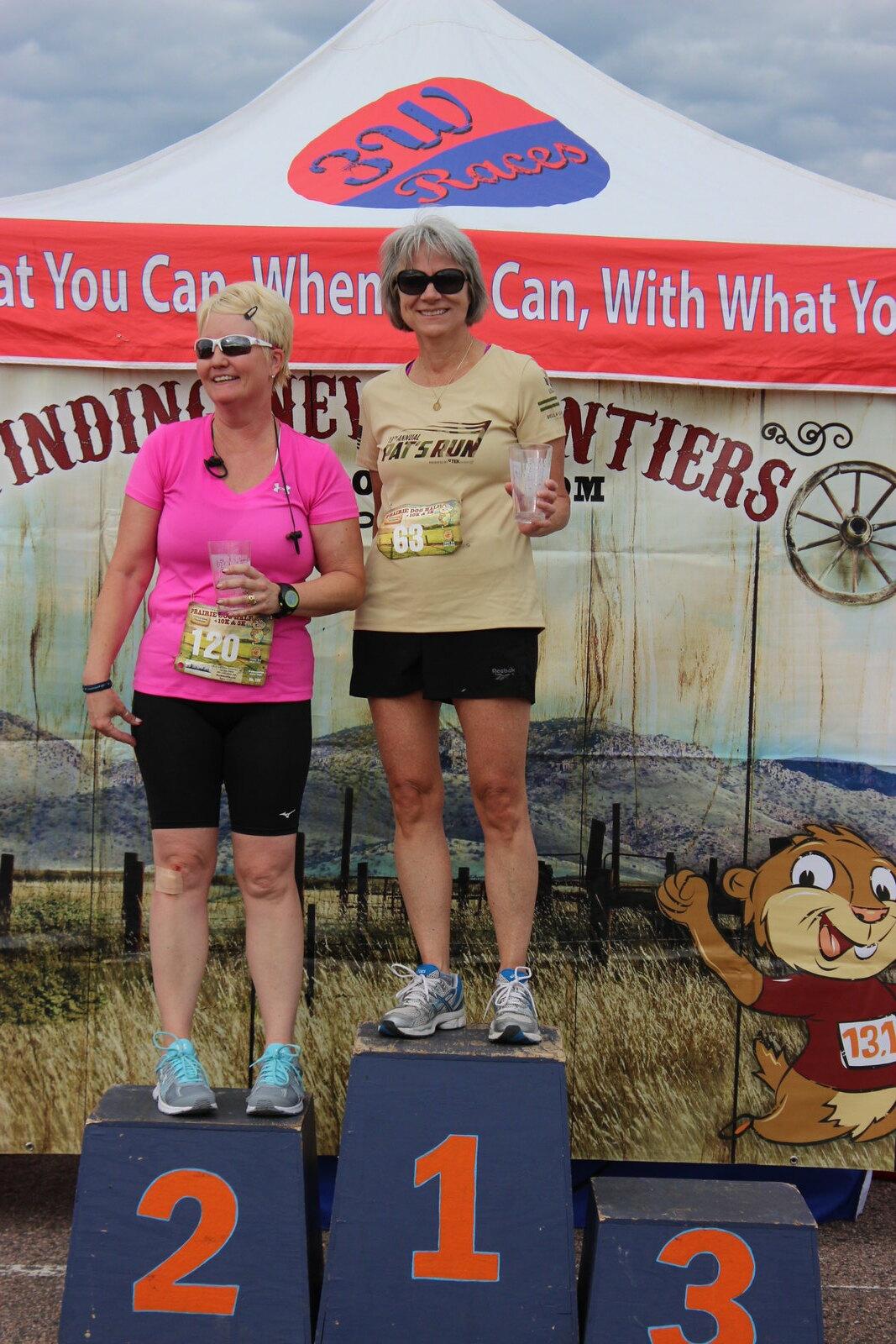In this vibrant outdoor color photograph, two women are standing on a navy-blue painted winner's podium labeled 1, 2, and 3, positioned against the backdrop of a large white tent with an orange border. Standing on box 1 to the right is a woman wearing a short-sleeved beige t-shirt, black shorts, sunglasses, and holding a glass in her left hand; she bears the bib number 63. To her left on box 2 is another woman dressed in a bright pink short-sleeved t-shirt, black shorts, white sunglasses, and also holding a glass in her left hand, with the bib number 120. Notably, the woman in second place has a band-aid on her right knee. Both women are wearing tennis shoes and appear to be dressed appropriately for a warm day. The third place box on the far right remains unoccupied. The scene is possibly from a running event, suggested by the bib numbers, with a mountainous terrain and a fenced field visible in the background, contributing to the picturesque and competitive atmosphere.